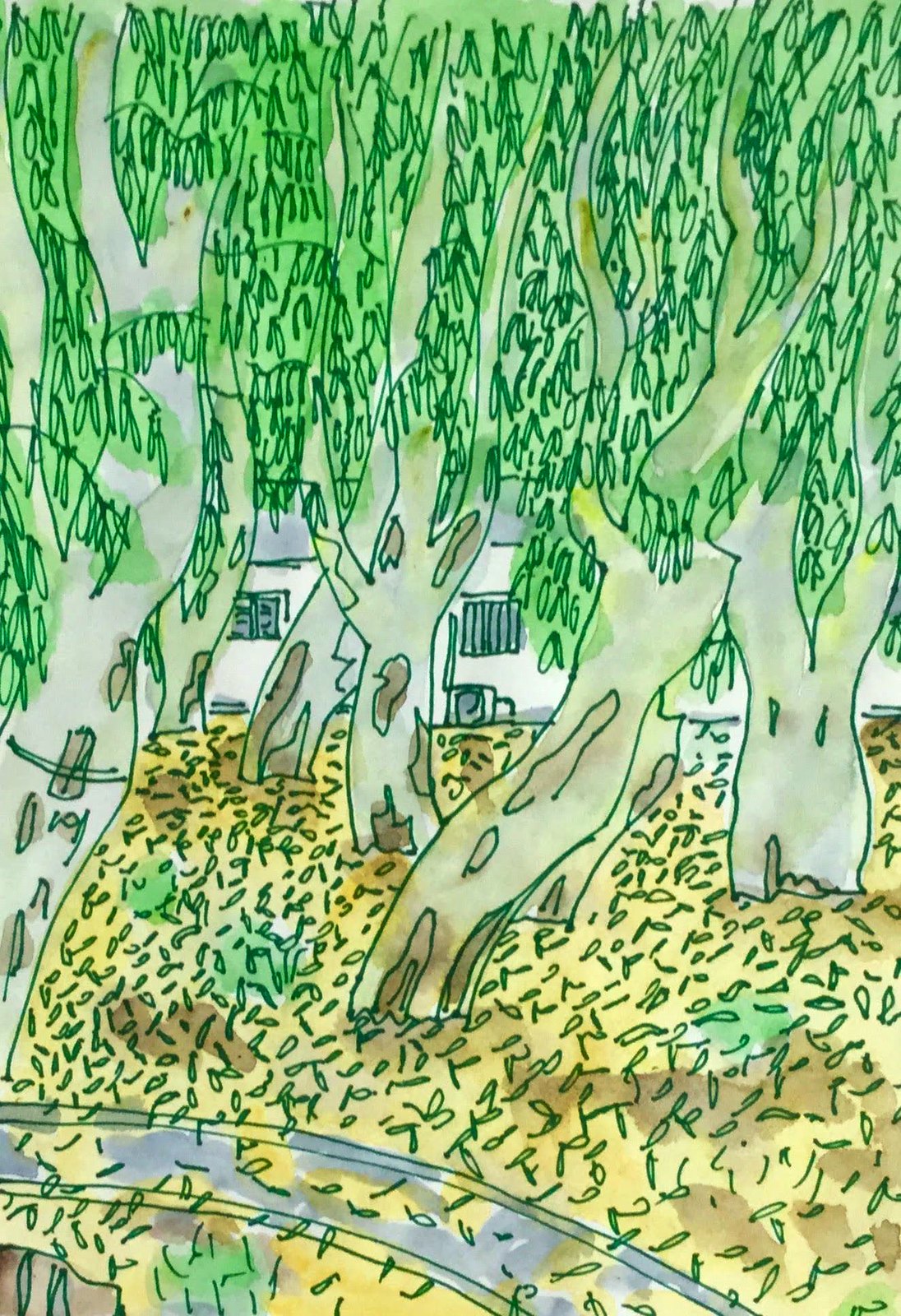This watercolor painting, rendered in a rectangular portrait orientation, beautifully captures a serene forest scene. The verdant green leaves of the trees contrast with their light gray and brown trunks, creating a sense of depth and tranquility. The forest floor is depicted in a harmonious blend of yellow, interspersed with spots of green, brown, and gray, suggesting a natural, untouched landscape. In the distance, partially obscured by the foliage, a quaint white house with a light gray roof and dark bluish-gray windows peeks through, adding an element of human presence amidst nature. Two distinct windows on the house are visible, anchoring the painting in a subtle yet poignant narrative.